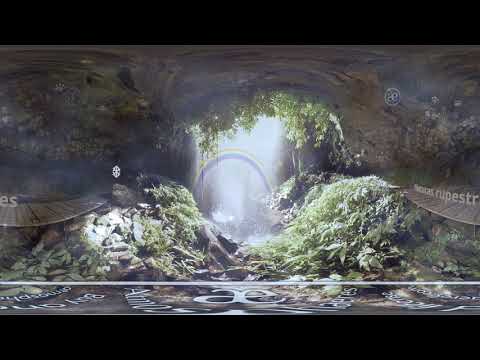The image showcases an interior view of a cave, captured with a fisheye lens, resulting in a curvy and warped perspective. Sunlight penetrates through an opening in the roof, creating a glowing central area. This bright spot is accentuated by a vivid rainbow with shades of red, yellow, blue, green, and purple, possibly hinting at a waterfall nearby. The cave's ceiling is a blend of brown and gray limestone rock, with green foliage dangling from above and flourishing on the ground below, giving the scene an almost rainforest or wetland ambiance.

On both sides of the image, you notice flat, wooden-looking walkways or platforms that might be man-made, leading through the cave. The overall atmosphere is hazy and ethereal, reinforcing the natural beauty of the environment. Additionally, there's some unreadable text along the bottom of the image featuring the letters “A-E” prominently, suggesting a logo or branding, possibly in a foreign language, adding a touch of modernity to the otherwise natural setting.